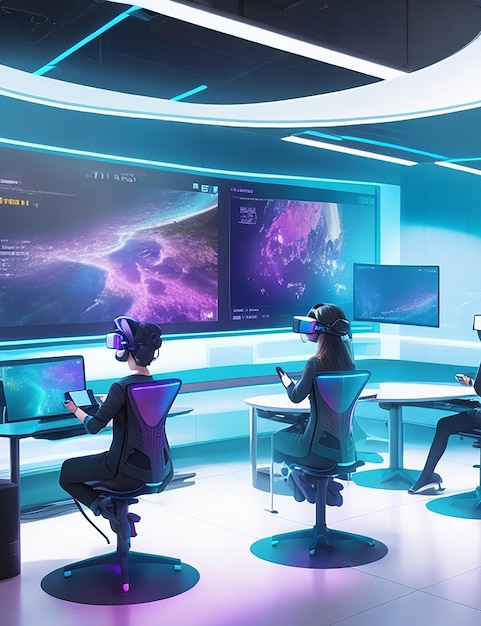The image is a digitally created illustration depicting a futuristic workspace with two people engaged in a virtual reality experience. Seated on sleek gray and silver desk or gaming chairs, both individuals wear dark-colored clothing and silver VR headsets that cover their eyes and most of their faces. The person on the left has short hair, sits at a desk with a large computer screen displaying a turquoise and purple backdrop, and holds a black handheld device with a small screen. The person on the right has long, dark brown hair, sits at a plain white table, and also holds a similar handheld device. The room is bathed in vibrant hues of blue and purple, with abstract, space-like purple and blue visuals on the wall in front of them. The setting features white floors and walls, with large, distinctive lighting fixtures on the ceiling, including both strip lights and a partially obscured, circular light. The entire scene exudes a high-tech, immersive atmosphere, blending elements of a modern office space with advanced virtual reality technology.